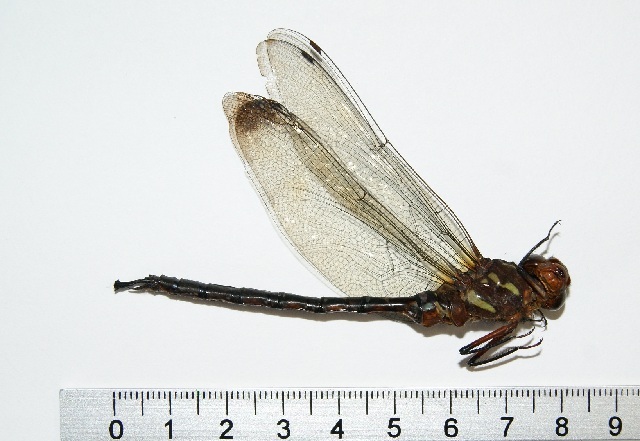The image shows a peculiar insect specimen that combines features of various bugs, resembling a hybrid with characteristics of a bee, centipede, and fly. Its most striking feature is its disproportionately large, almost clear wings, which are bigger than its body. The body, particularly the tail section, is very dark in color, predominantly brown and deep hues. The insect lies on a table, with its entire length measured by a ruler placed below, indicating it is approximately eight to eight and a half inches long. The ruler, marked from zero to nine, ascends from left to right, matching the orientation of the insect, which is also positioned from left to right and facing rightwards. Visible details include curled-up legs, antennas on its head, and distinguishable eyes. The setting suggests a scientific or educational environment, possibly for the purpose of studying and presenting the specimen for academic purposes.